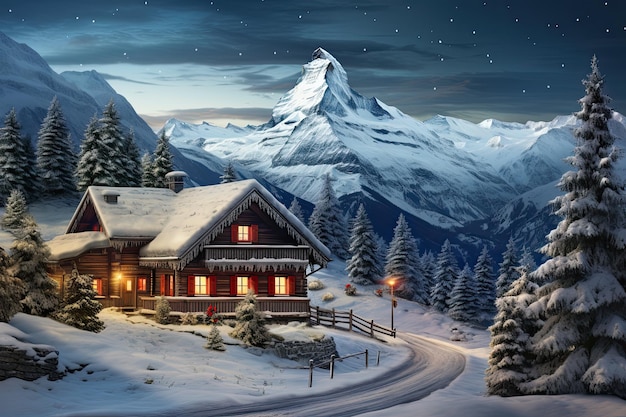The scene, which evokes the sentimental style of Thomas Kinkade, features a cozy cabin nestled in a snowy, mountainous landscape. On the left, a charming chalet with a pointed roof stands adorned with snow and warm lights glowing from multiple windows. The upper porch has a single window, while the wraparound lower porch shows three windows on the viewer's side, two more around the corner, and a door facing forward. Two chimneys rise from the roof, and a wooden fence surrounds the property. On the right-hand side of the image, an extra-large, snow-covered tree accompanied by a smaller tree stands prominently. In the background, majestic, snow-capped mountains extend beneath a dark sky speckled with stars. A slightly cleared, curving street cuts through the scene, bringing life to the quaint, moonlit landscape. A streetlight near the fence contributes to the inviting, serene atmosphere of this picturesque winter night.